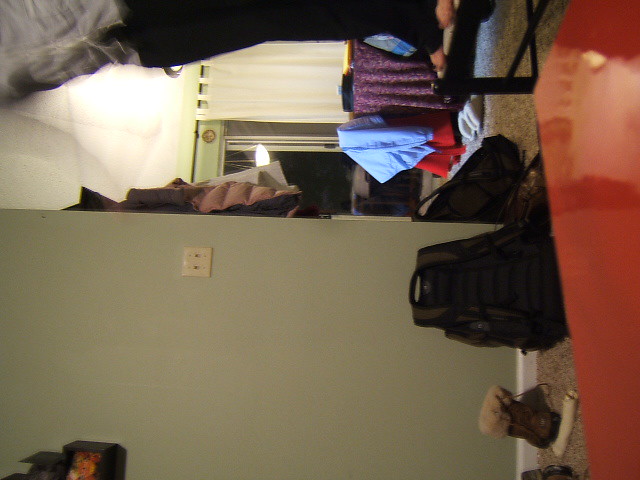In this sideways photograph of a cluttered living room leading into a dining area, we see a person standing on a black chair. They are dressed in dark pants with a tag visible, orange socks, and a white shirt. The room has green walls and brown carpet. The person has removed their boots, which are seen next to a black backpack resting against the off-green wall. A table covered with a tablecloth, which appears to be purple or maybe blue with a red piece of cloth on it, is visible. A sliding glass door with drapes hanging over a bar is also featured. Additional items in the image include a coat rack with a coat above a wooden console, curtains, a light switch with two switches, and a pair of slippers. The entire right side of the picture is dominated by what looks like a red coffee table.